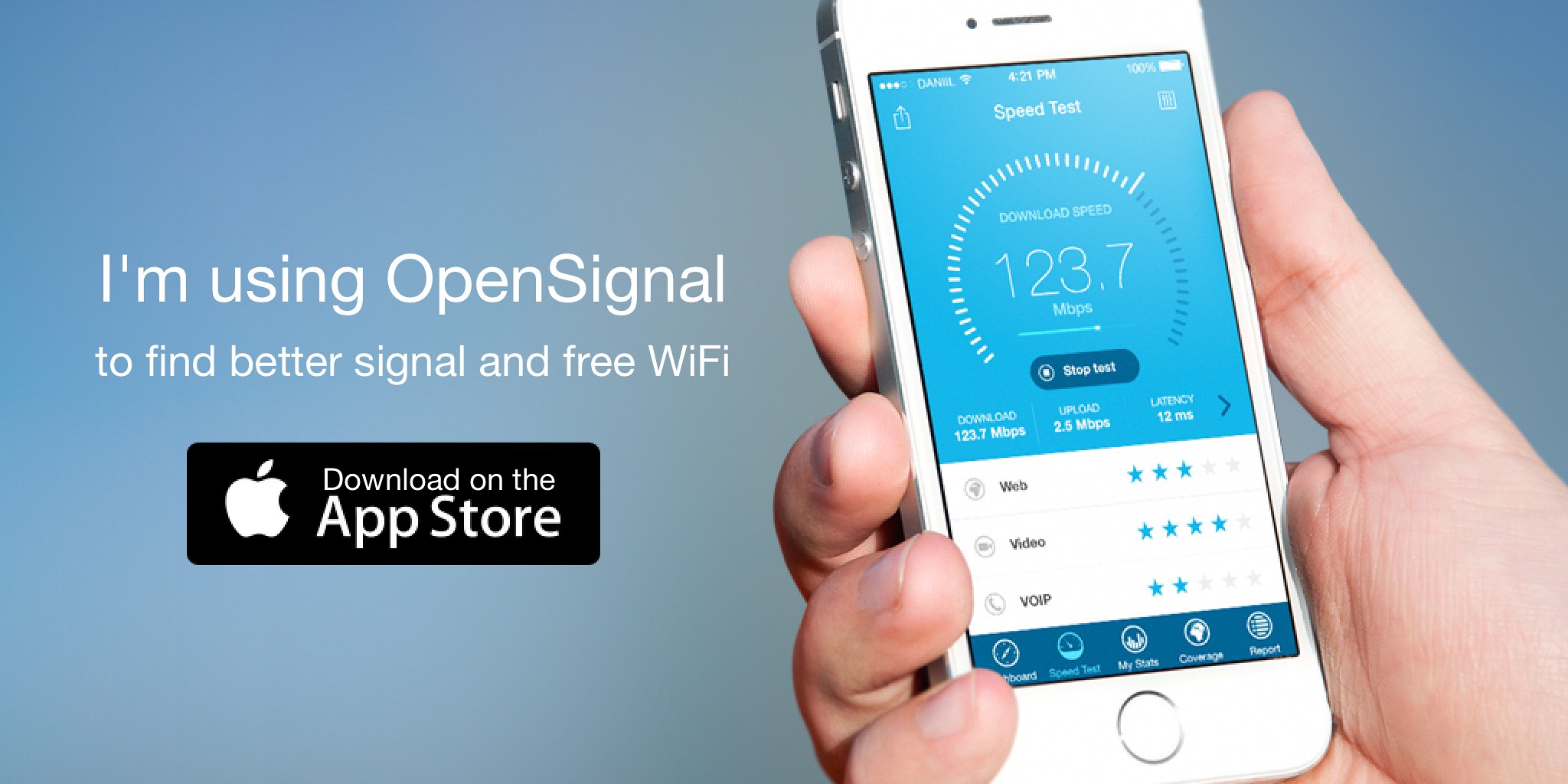This is a rectangular, horizontal print advertisement for an app called OpenSignal. The main colors used are white, blue, and black. The right side of the image features a white person's right hand holding an older iPhone, displaying the OpenSignal app. The iPhone's screen has a blue background and shows a speed test with the following results: download speed of 123.7 megabits per second, upload speed of 2.5 megabits per second, and a latency of 12 milliseconds. Below the speed test results, there are star ratings for different types of internet usage: two blue stars for Voice over IP (VoIP), four blue stars for video, and three blue stars for web. 

On the left side of the image, in white text, it reads, "I'm using OpenSignal to find better signal and free Wi-Fi." Below this, in a black rectangular bar with white text, it says, "Download on the App Store," accompanied by the iconic Apple logo. The overall design highlights the app interface and its features, emphasizing the benefits of using OpenSignal to improve signal strength and locate free Wi-Fi.